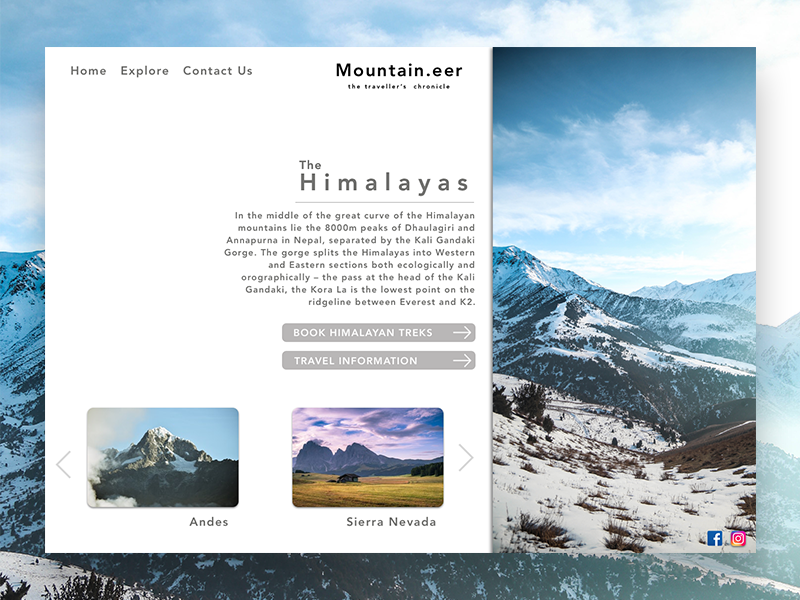This is an image of a webpage dedicated to the Himalayas, featuring a detailed pop-up overlay. The entire background of the page displays a breathtaking view of the Himalayan mountain range, characterized by snow-covered peaks and patches of grassy areas interspersed with twigs. 

In the bottom right corner of the image, there are icons for Facebook (denoted by an 'F') and Instagram, indicating options for social media sharing. At the top of the webpage, a navigation menu provides links with labels such as 'Home,' 'Explore,' 'Contact Us,' and 'Mountain Ear' (stylized as mountain.eer), which is associated with 'The Traveler's Chronicle.'

Prominently displayed on the page is a section titled "The Himalayas," which states: "In the middle of the great curve of the Himalayan mountains lie the 8,000 peaks of Dhalagiri and Annapurna in Nepal, separated by the Kali-Gandaki Gorge. The gorge splits the Himalayas into western and eastern sections both ecologically and orographically. The paths at the head of the Kali-Gandaki and the Karli rivers represent the lowest point on the ridgeline between Everest and K2."